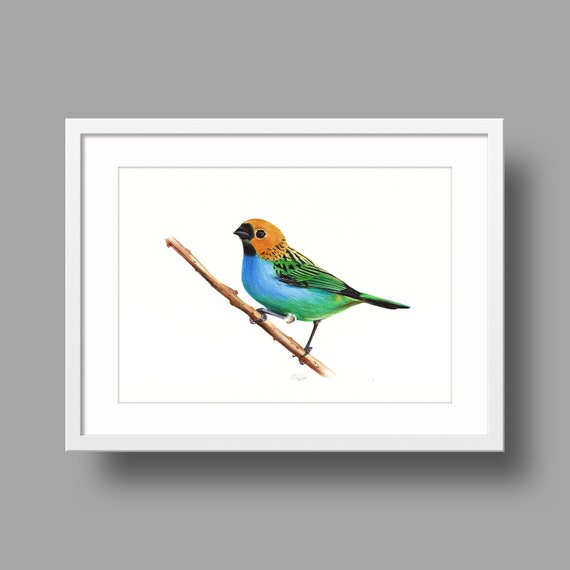Displayed within a white square frame, mounted on a medium gray wall, is a watercolor painting of a vibrantly colored, small-sized bird. The bird stands on a branch positioned at a 45-degree angle. This avian subject features a blue chest and belly, with green on its underside, and green and black feathers on its wings. The bird has an orange head adorned with a black spot just below its black beak. The minimalistic background accentuates the bird's vivid colors and detailed portrayal, emphasizing its presence. No text accompanies the image, drawing complete focus to the intricately painted bird.